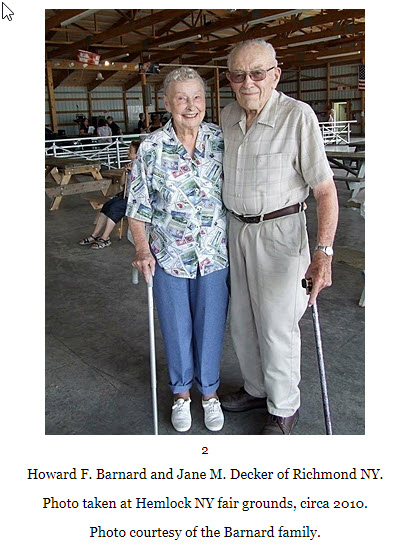The photograph captures a candid moment of two elderly individuals, Howard F. Barnard and Jane M. Decker of Richmond, New York, posing indoors at the Hemlock, New York, Fairgrounds around 2010. Howard is dressed in a brown plaid shirt, khaki pants fastened with a dark brown belt, brown shoes, and a wristwatch. He is balding and wears glasses, his cane held in his left hand. Beside him stands Jane, clad in a white shirt adorned with blue illustrations resembling postcards, paired with blue pants and white sneakers. She grasps a cane in her right hand. The setting features a dirt ground, with a woman seated at a picnic bench or chair in the background. The enclosing space suggests a hall with visible rafters, walls, lights, and a fence, giving it a rustic, fairground feel. A mouse cursor is visible on the left side of the photograph, indicating it was captured as a screenshot. The caption below the image states: "To Howard F. Barnard and Jane M. Decker of Richmond, New York. Photo taken at Hemlock, New York, Fairgrounds, circa 2010. Photo courtesy of the Barnard family."